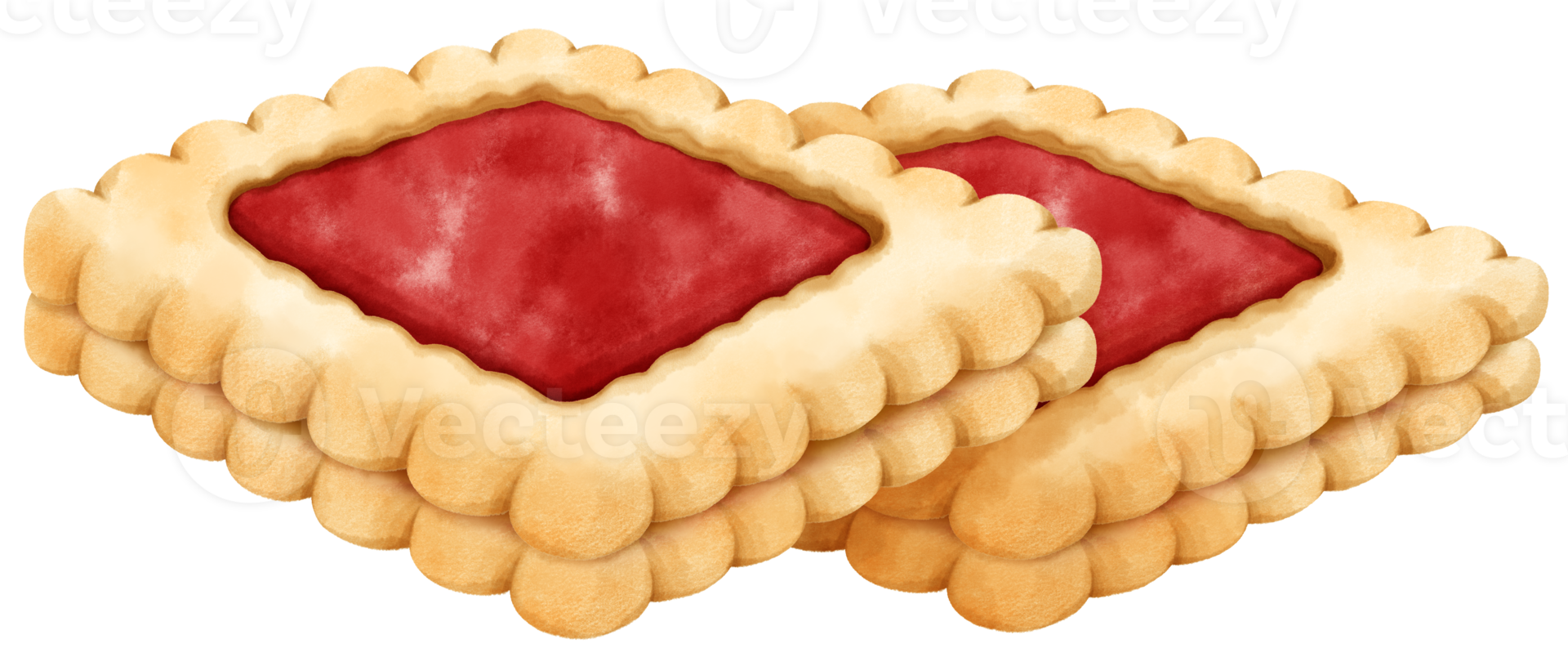The image showcases a highly realistic watercolor painting illustration of two large, fancy shortbread cookies. These sandwich-style cookies have a unique square or rectangular shape with intricately fluted edges. Each cookie is composed of two layers and features a smaller, square cutout in the center that is filled with vibrant red jelly. One cookie is artfully stacked on top of the other, making their structure and details prominent. The background of the image is transparent, devoid of any distractions. A watermark reading "Vecteezy" appears four times across the photo, partially transparent at around 20% opacity, signifying its affiliation with a stock photo source. This detailed and elegant depiction makes it challenging to decipher whether it's an actual photo or a masterfully created drawing.